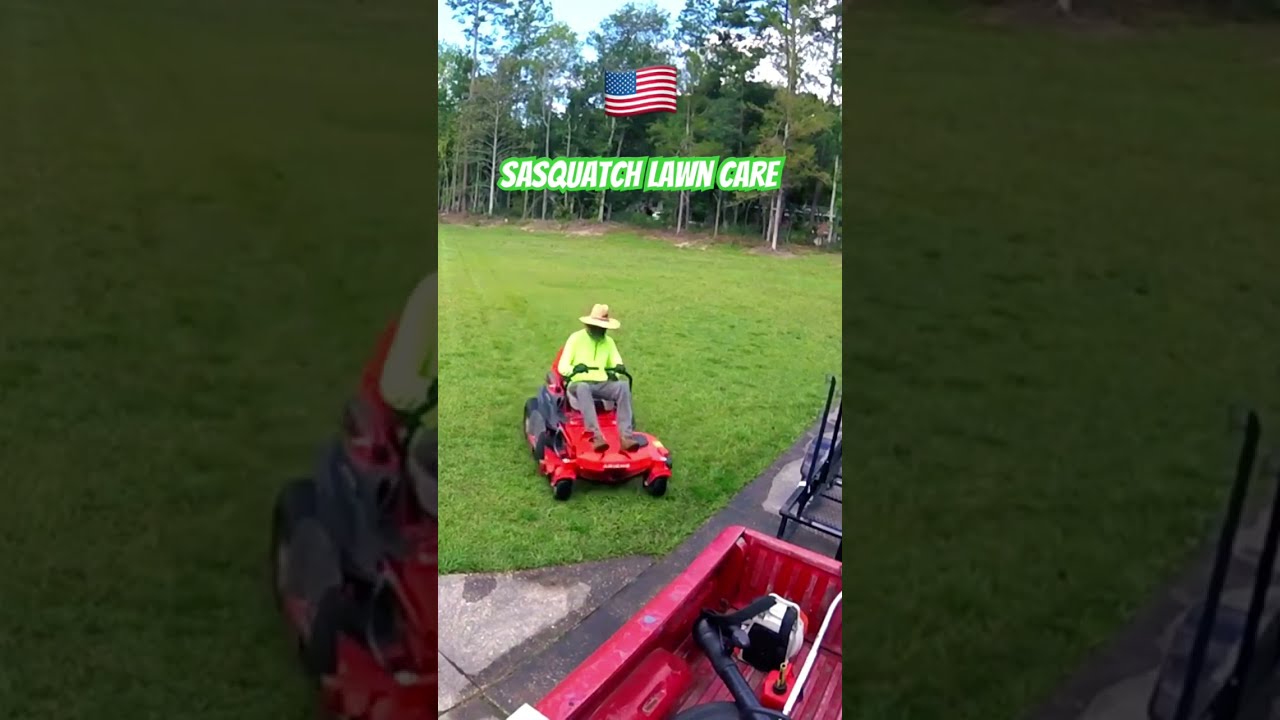This detailed image captures a vibrant outdoor scene in the middle of the day, featuring a man centrally located on a lush green lawn, riding a red lawnmower. The man is dressed in a beige hat, light green shirt, and gray pants. Behind him, a sign reading "Sasquatch Lawn Care" is prominently displayed, with the bold green letters having white interiors. Above the sign waves an American flag with blue, white, and red stripes. 

In the background, tall, thinly-leaved trees suggest a spring setting, with a hint of sky visible above. From the bottom of the image, you can see part of a truck or trailer, a wheelbarrow, and the slightly peeking edge of a sidewalk and pavement, forming a triangular visual with the truck and a trailer that contains yard tools, including a leaf blower.

This image is horizontally rectangular, where the central vibrant image is bordered on the left and right by faded close-up segments of the scene, providing a wider context while maintaining focus on the man mowing the lawn. The overall setting, combined with the overlay style, suggests that it could be a screenshot from a social media app like TikTok or Instagram Live.